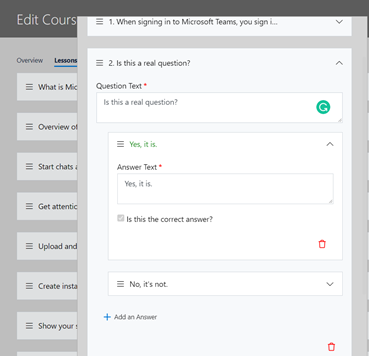This image is a cropped screenshot of an educational application, likely running on a tablet or PC based on its resolution and shape. The interface appears to be part of a course management system, as indicated by the partially visible background text "edit course," which is cut off at the "S." The visible portion of the application shows a list of clickable white options, such as "MIC," "overview of stat charts," among others. The highlighted section, labeled "lessons," is underlined in blue, suggesting it is the currently active category, indicating it might be part of a school course structure.

In the primary window at the top, there is a partially visible issue report related to Microsoft Teams; the text begins with "when signing into Microsoft Teams, you sign in and then," followed by a cutoff, with the word "two" visible beneath it. This text seems to be associated with a question creation feature. A prompt asks, "Is this a real question?" with the selectable answer, "Yes, it is," suggesting that users can create and edit questions for courses. This tool appears to facilitate the development of tests or quizzes that students can complete.